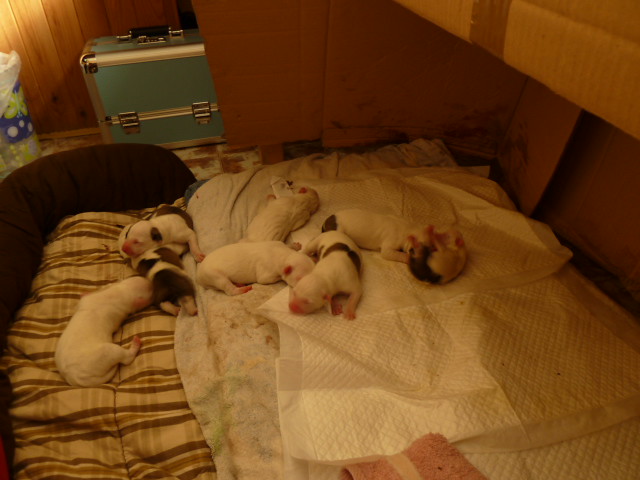This indoor color photograph, taken under artificial light with a yellowish overcast tinge, captures a litter of newborn puppies, likely only a few days old, sleeping on a makeshift bed. The bed is composed of a white training pad, a striped blanket, a lighter green and cream floral quilt, and a very light cream one with an embossed design. The puppies, numbering eight in total, are various shades of white, black and white, and white with black stripes or splotches. They have pink ears, noses, and feet, and seem to be sleeping soundly with their eyes closed, curled up closely together. Their resting area appears to be a combination of sheets and duvet covers, surrounded by a wooden structure with visible walls at the back and side, and possibly a ledge in the upper right corner. To the left, there is a noticeable black edge, suggesting they might be on a pull-out couch. In the upper left corner, there's a metallic-edged green case with padlocks, a white bin or kitchen roll with a green and blue label, and a light source that's brighter than the rest of the scene. Additionally, there's a hint of a blue metallic suitcase in the background and a cardboard box adjacent to what appears to be a doggie bed on the left.